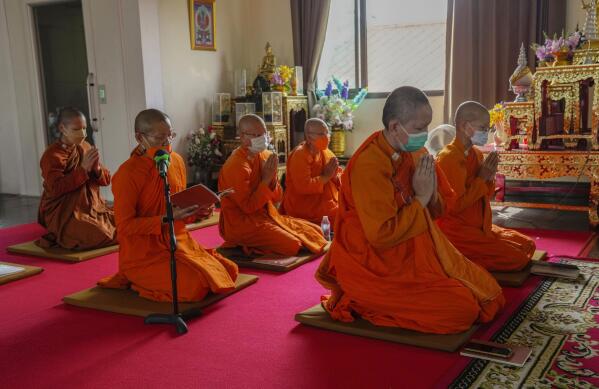The image captures a serene moment inside a Buddhist temple, where six monks clad in deep orange robes are kneeling on prayer mats atop a red carpet. All of them are wearing face masks, reflecting a time possibly during the pandemic. The monks, many of whom are bald and some wearing glasses, are arranged in three rows, with their hands clasped in prayer. One monk in the middle section holds a red book and has a microphone close to their mouth, likely reciting prayers or chants. On the right side of the image stands an ornate gold shrine adorned with colorful flowers, with a gold Buddha statue perched at the top. The shrine is positioned beside a partially open window with brown curtains, allowing daylight to cascade in. A patterned carpet can also be glimpsed in front of the monks, adding to the temple's rich, sacred decor.